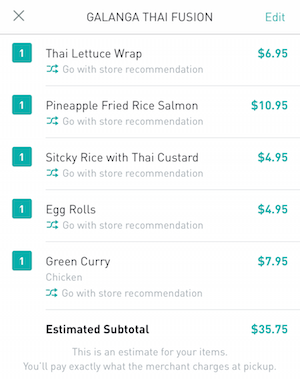The image displays a detailed menu from Galanga Thai Fusion, showcasing a customer's recent pickup order totaling $35.75. The ordered items include one Thai Lettuce Wrap, Pineapple Fried Rice with Salmon, Sticky Rice with Thai Custard, Egg Rolls, and Green Curry. The menu is presented on a white background with black text and features greenish design elements. It also notes that the subtotal is estimated, emphasizing that the final amount paid will align with the merchant's charges at pickup. The most expensive item is the Pineapple Fried Rice with Salmon, while the least expensive are the Sticky Rice with Thai Custard and Egg Rolls.